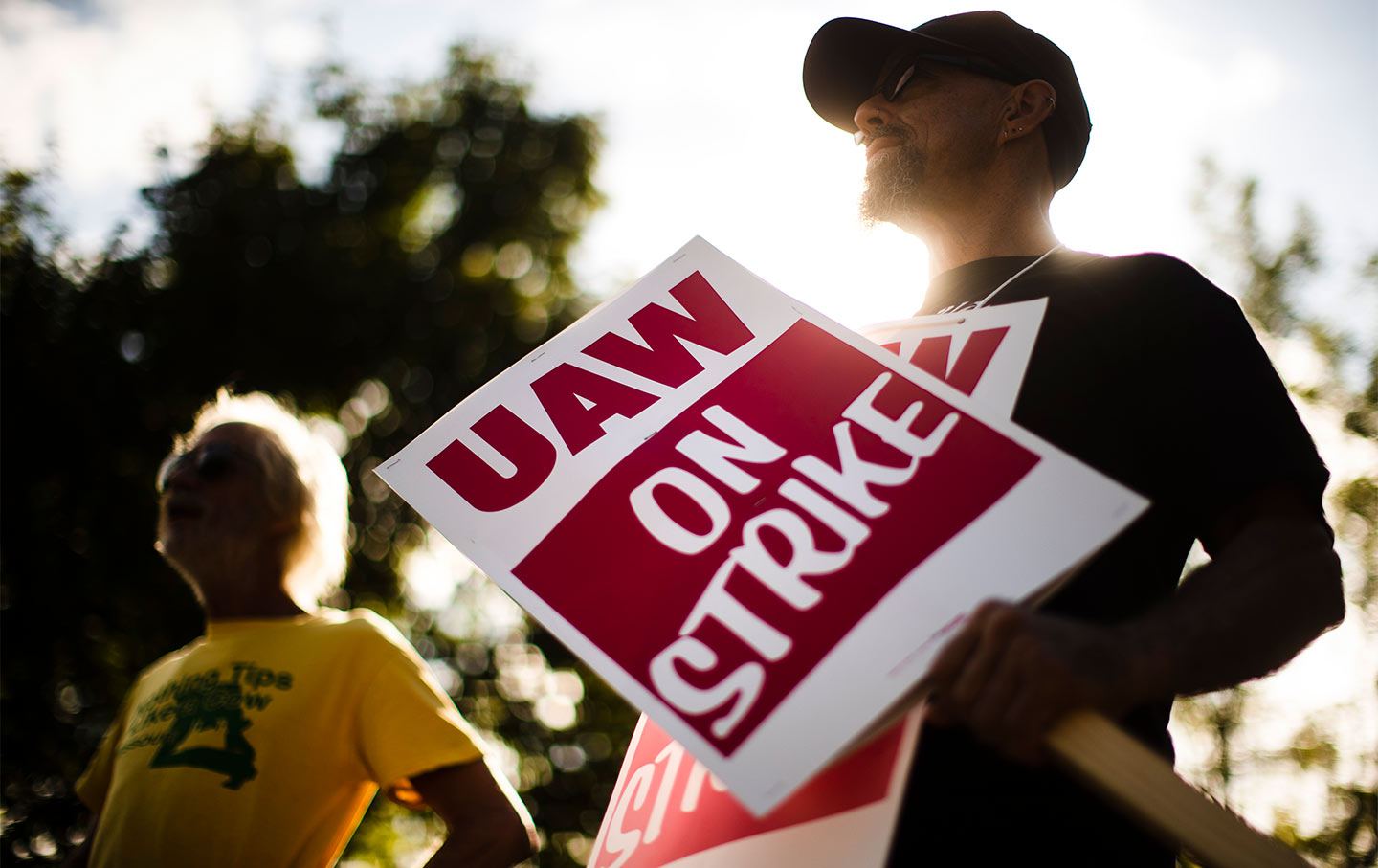This outdoor photograph features two men standing in the foreground against a slightly hazy backdrop, suggesting a sunny day with a blue sky and some scattered clouds. Tall, bright green trees and foliage frame the scene, adding vibrancy to the setting. 

On the left side of the image stands an older, tan white man with white hair and a beard. He sports black sunglasses and wears a yellow t-shirt with a forest green logo and text, details of which are not clearly visible due to the small size. 

Dominating the right side of the photo is a middle-aged white man with a black baseball cap and sunglasses. He has multiple piercings—ear and nose—a closely trimmed salt-and-pepper mustache and goatee, and dons a long-sleeve black t-shirt. Around his neck is a sign tied with a string. He is also holding a protest sign attached to a wooden stick which prominently displays the words "UAW on strike" in red and white lettering. 

The overall composition highlights these two individuals, with the man on the right, who appears ready for a demonstration or rally, being the primary focus given his distinctive attire and signs.